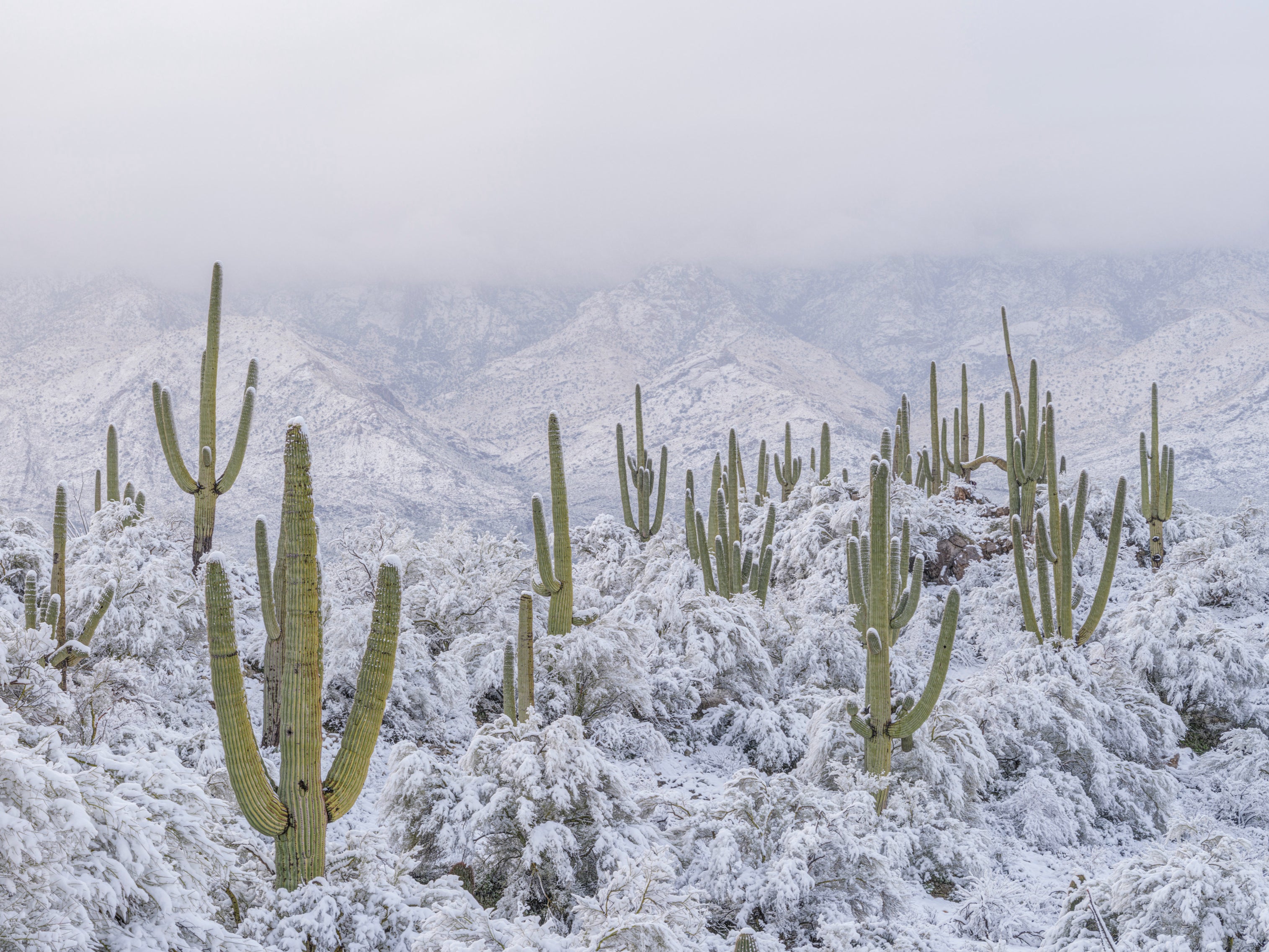This photograph captures a rare and remarkable winter scene of a desert landscape covered in snow. In the foreground, tall, green cacti rise prominently from the ground, surrounded by low, dried bushes, and desert scrub all blanketed in a light dusting of snow. The terrain is hilly and uneven, adding texture and depth to the scene. As the eye moves toward the background, a range of rugged, snow-covered mountains stretches across the horizon, capped by a thick, foggy sky. Heavy clouds hover low over the mountains, creating a stark contrast with the unusual snowy desert terrain below. Despite the dense cloud cover, the image is illuminated by daylight, highlighting the surreal beauty of the snowy desert and the large, overgrown cacti that dot the landscape.